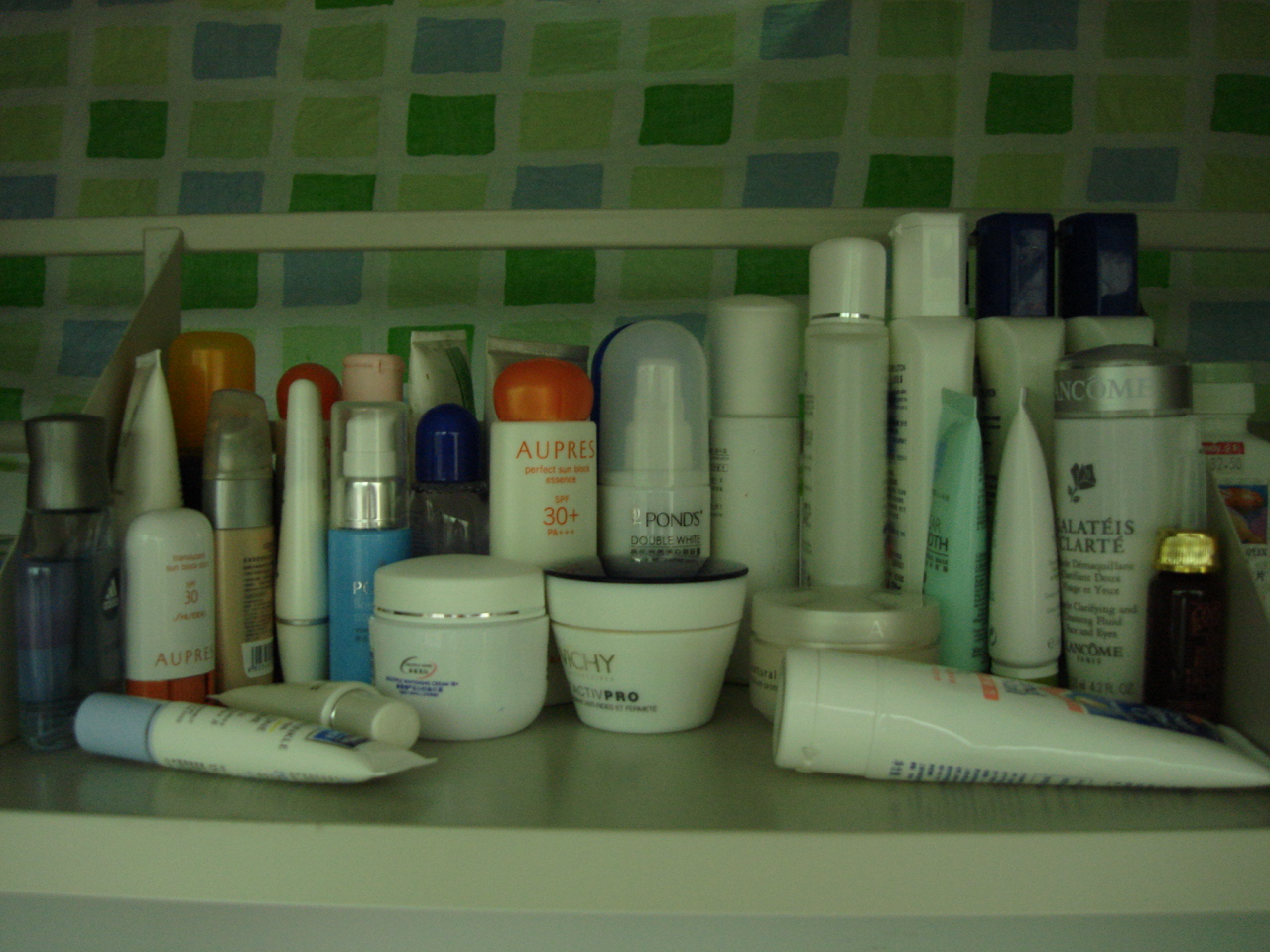In this vibrant and meticulously organized photograph, a lady's extensive collection of beauty products is displayed on an approximately 8-inch deep shelf. The shelf is densely populated with a diverse array of lotions, creams, and sprays, reflecting a comprehensive skincare and beauty regimen.

The backdrop features a colorful checkerboard pattern that adds a lively touch to the scene, with alternating blue, yellow, green, and red squares. This decorative element could be either a tiled wall or a patterned towel or sheet, enhancing the visual richness of the setup.

Among the myriad of products, two items prominently display the brand name "AUPRES". A bottle with a spray top from Pond's can also be seen, adding to the variety. There are three wide jars with lids, likely containing moisturizing creams, hinting at a focus on skincare. Numerous other bottles and tubes, potentially for shampoos and conditioners, fill the remaining space. One can also spot products from the renowned brand Lancôme, further emphasizing the diversity and luxury of the collection.

The scene is a testament to the meticulous care and attention that goes into maintaining such a formidable assortment of beauty products.